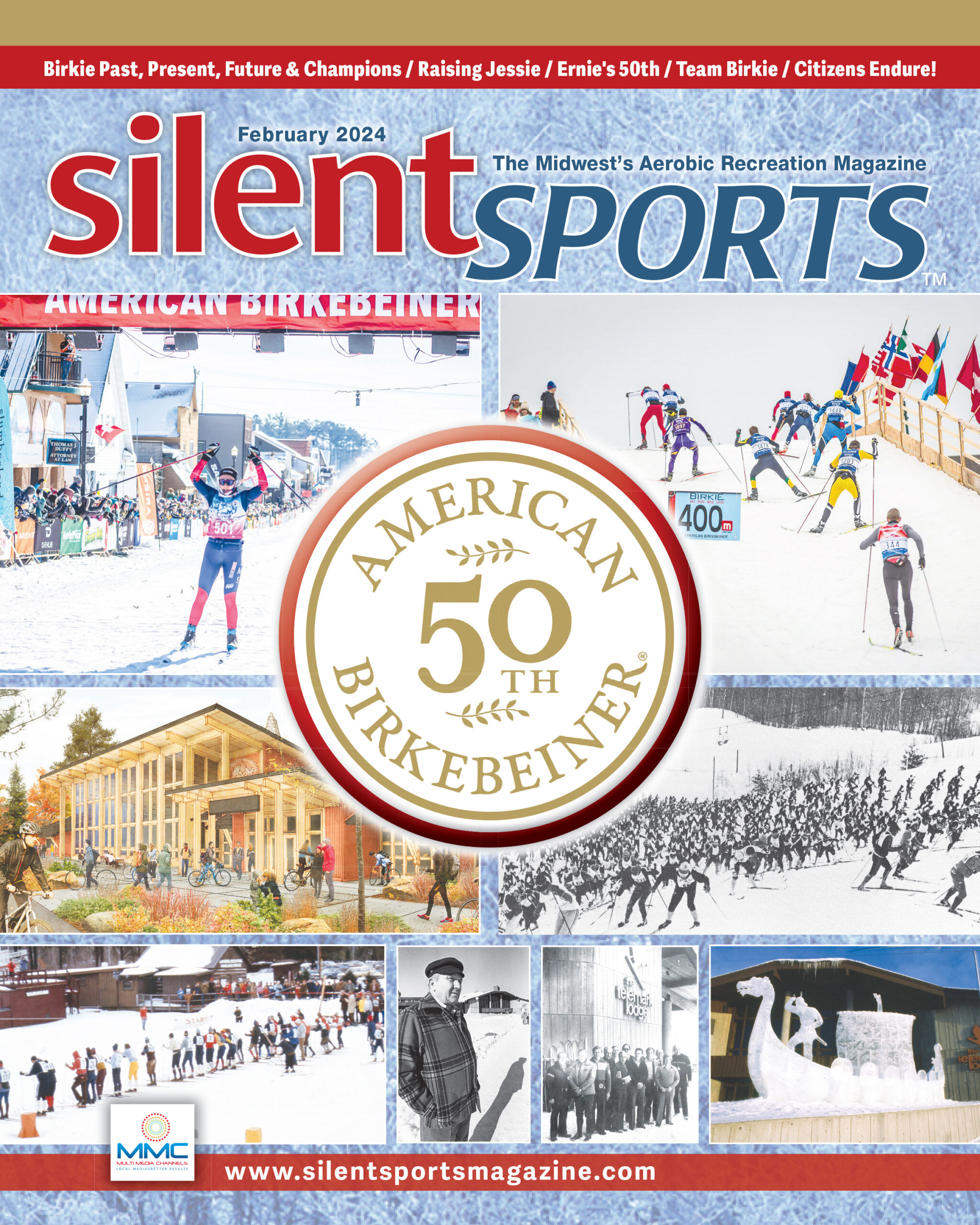The magazine cover, dated February 2024, features the title "Silent Sports: The Midwest Aerobic Recreation Magazine" prominently at the top. The upper section of the cover is divided into a gold bar followed by a red bar with white text listing key articles: "Berkey Past, Present, Future," "Pan Am Champions," "Raising Jesse," "Ernie's 50th," "Team Berkey," and "Citizens Endure." Below this header, the background features a picturesque winter scene with snow-covered trees.

Centered on the cover is a circular emblem with gold text reading "American 50th Berkbiner," encased in a red circle, adding a focal point to the design. Surrounding the emblem are various images depicting winter sports enthusiasts. There are scenes of individuals skiing, including a busy snapshot of people downhill skiing and a photo of a golden-colored building that appears to be a ski lodge with a snow-covered hill in the background. Additional pictures show people in line on skis, a man in a coat, a group of unidentified individuals, and what appears to be a boat icicle.

The cover also includes the magazine's website, www.silentsportsmagazine.com, along with the description "The Midwest Aerobic Recreation Magazine" positioned strategically to attract readers interested in winter sports and activities.